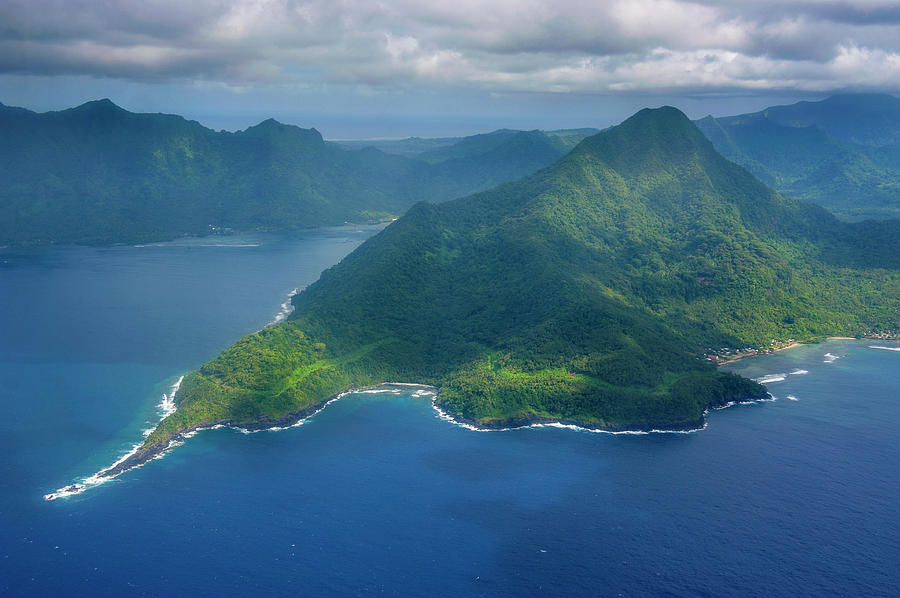A breathtaking aerial photograph captures a stunning tropical island and its surrounding waters beneath a sky filled with an array of clouds—ranging from fluffy white to darker storm-like grays. The island is densely covered in lush, vibrant greenery with various shades of green influenced by the cloud cover. 

In the middle left, a mountain range with distinct peaks extends downward in a pointed tail-like formation. A broader mountain range traverses the image from left to right, adding grandeur to the scene. There are visible shades of dark green across these mountains, interspersed with lighter green areas. 

The ocean surrounding the island is a deep, dark blue, significantly darker than the sky, with variations in blue hues. Near the edges of the island, the water becomes clearer, and small beach areas with sandy shores are visible, with waves crashing gently along the coastlines. The scene captures a few distinctive extras—a small harbor with tiny white boats on the right, and what might be homes or structures on the shore, adding a hint of human presence to the otherwise remote and lush landscape.